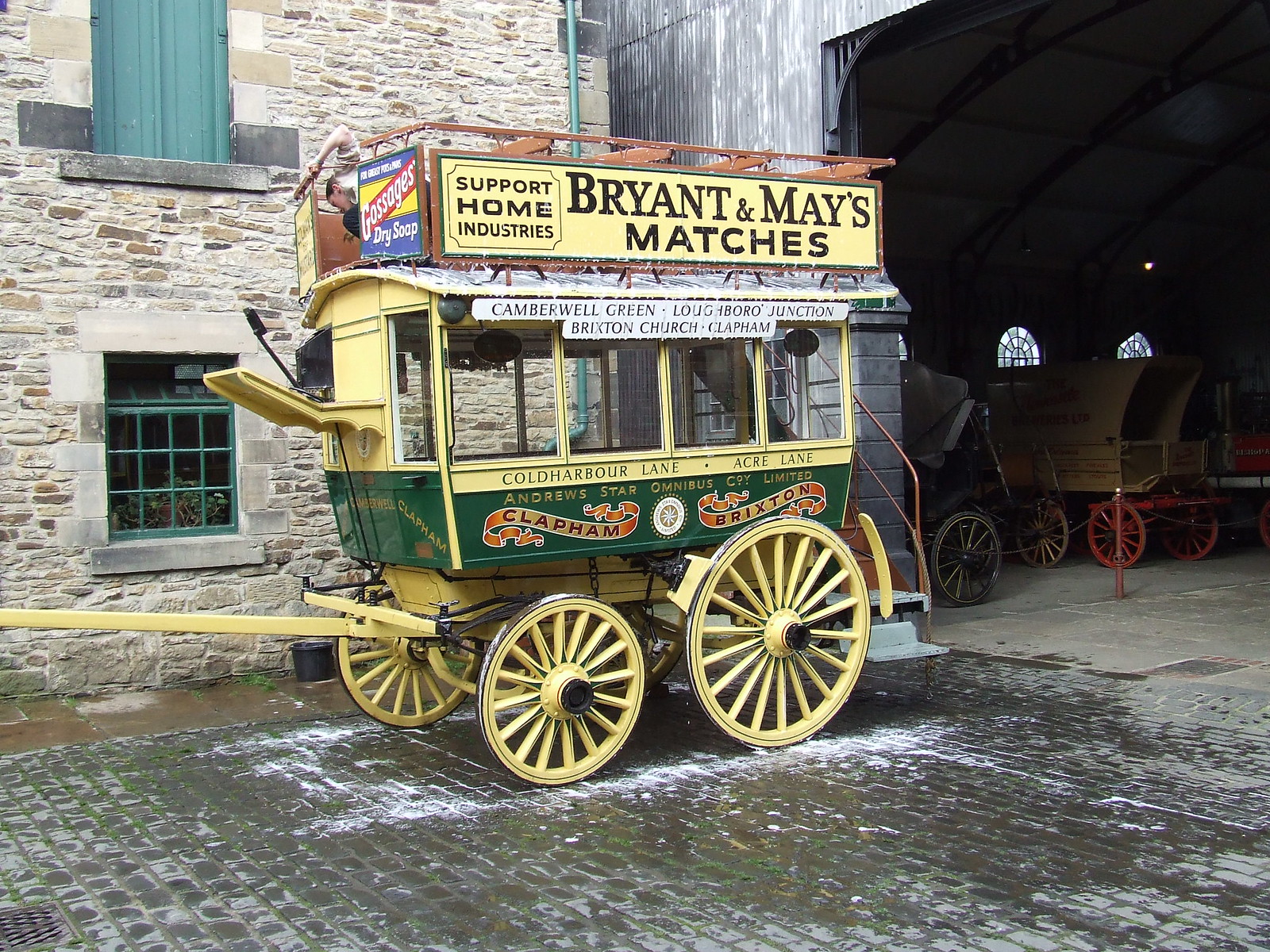This image captures a picturesque scene in front of an older, light gray and brown cobblestone building. The building, which extends upwards beyond the image's frame, features green window frames and lush green curtains. In the foreground, an old-fashioned carriage is prominently displayed. Painted in vibrant shades of green and yellow, the carriage bears several advertisements: "Bryant and May's Matches" is emblazed at the top in black on a yellow banner, "Support Home Industries" on the left side, and locations such as "Camberwell Green, Loughborough Junction, Brixton Church, Clapham" are listed below hanging from the windows. The carriage boasts windows around its sides and has two smaller yellow-spoked wheels at the front and two larger ones at the back. To the right, inside a shadowy barn, several other carriages can be seen, some with black wheels and others with red. The setting reflects a charming, nostalgic atmosphere, echoing the bygone era of horse-drawn transportation.